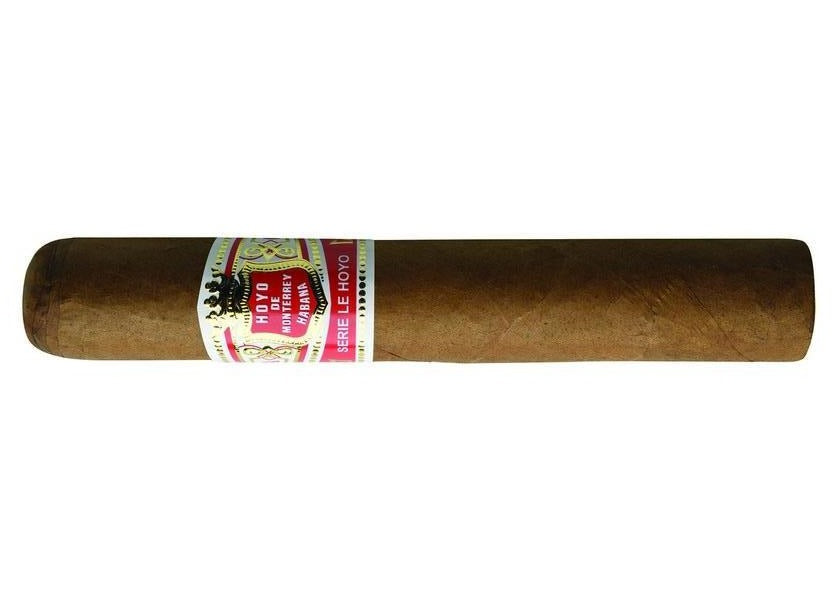This close-up image showcases a single, horizontally arranged cigar, carefully placed on a blank white background, emphasizing its elegant appearance. The cigar is long and tightly wrapped in a light brown leaf, with the rounded end on the left and the lit end on the right, slightly darker in shade. The focal point is the ornate label wrapped around its center, which reads "Hoyo de Monterrey Habana" in an all-caps white font. The label, predominantly white with gold and red accents, presents a regal and royal aesthetic. The central red crest, adorned with a golden crown, adds to its prestigious look, accompanied by red banners and golden dots. The image resembles an advertisement, meticulously edited to highlight the cigar’s luxurious and premium branding.